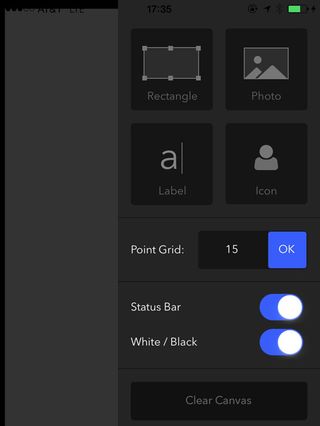The image is a vertically-oriented screenshot, likely captured from a smart device's screen. The background is a seamless blend of solid black and dark gray colors with no discernible texture, creating a subtle gradient effect. 

On the top left of the screen, a series of small icons are visible—signal bars, the "AT&T LTE" network indicator, and the time displayed in military format: 17:35. Adjacent to these, a set of symbols including a circular icon, possibly for location services, a Bluetooth symbol, and the battery indicator show a green color, suggesting the device is charging.

The main area of the screen features several black rectangular boxes overlaid on the gray background. Each box contains different elements: one is a plain rectangle, another displays a photo, the third has the letter "A" with a vertical line labeled "label", and the fourth box contains an outline of a person icon labeled "icon".

Below these, the interface displays options related to a point grid system, showing "15" and an "OK" button in blue. Further options indicate toggles for "status bar" and a "white/black" feature, both turned on. At the very bottom of the screen, there is a "clear canvas" button, indicating an action that can be performed.